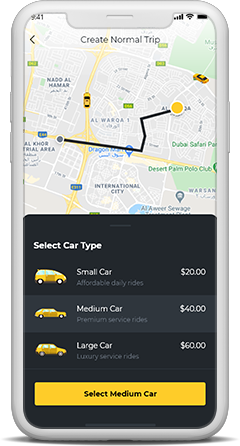A white smartphone, resembling an iPhone, displays a ride-sharing app interface. The screen's upper half shows a map peppered with small yellow car icons, labeled "Create Normal Trip" above it. The lower half of the screen features a black backdrop with the text "Select Car Type." This section presents three car options: 

1. A "Small Car" described as "affordable daily rides" priced at $20.
2. A "Medium Car" labeled as "premium service rides" priced at $40.
3. A "Large Car" offering "luxury service rides" at $60.

Beneath the car options, a prominent yellow bar reads "Select Medium Car."